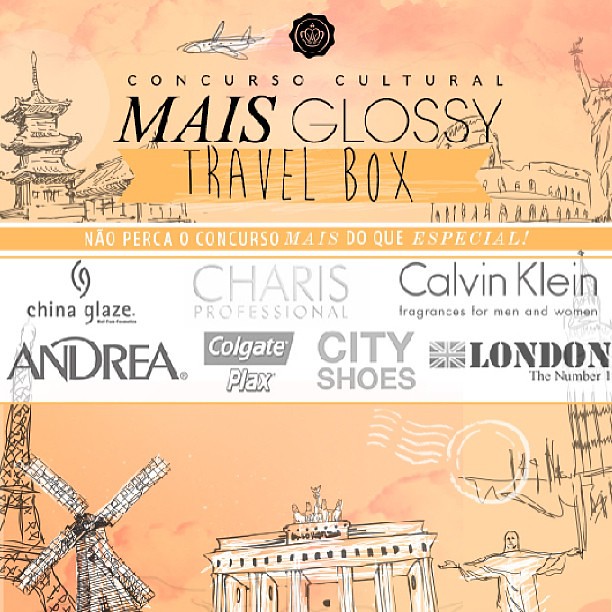The image showcases an advertisement for a promotional item labeled "Concurso Cultural Mais Glossy Travel Box." The packaging features a detailed, illustrated design that spotlights various global landmarks against a peach-colored background with a watercolor texture. At the very top, a jet plane is depicted soaring across a light orange sky. Underneath, the top section includes illustrations of notable landmarks such as the Roman Colosseum, the Statue of Liberty, and traditional Chinese architecture. The text "Concurso Cultural Mais Glossy Travel Box" appears prominently in black letters. 

In the middle section, a white banner lists several brand logos, including China Glaze, Andrea, Colgate Plaques, Shiree's Professional City Shoes, Calvin Klein, and London No. 1, all rendered in gray and black letters. 

The bottom section returns to the light orange background, where additional landmarks are illustrated: the Eiffel Tower, a windmill, Christ the Redeemer statue in Rio de Janeiro, and a classical structure with columns and statues on top. The landmarks are dispersed across the packaging, creating an appealing blend of culture and travel. The vivid visual presentation emphasizes the theme of travel, with a palette that melds warm peach tones with pink hues to evoke a sense of adventure and discovery.